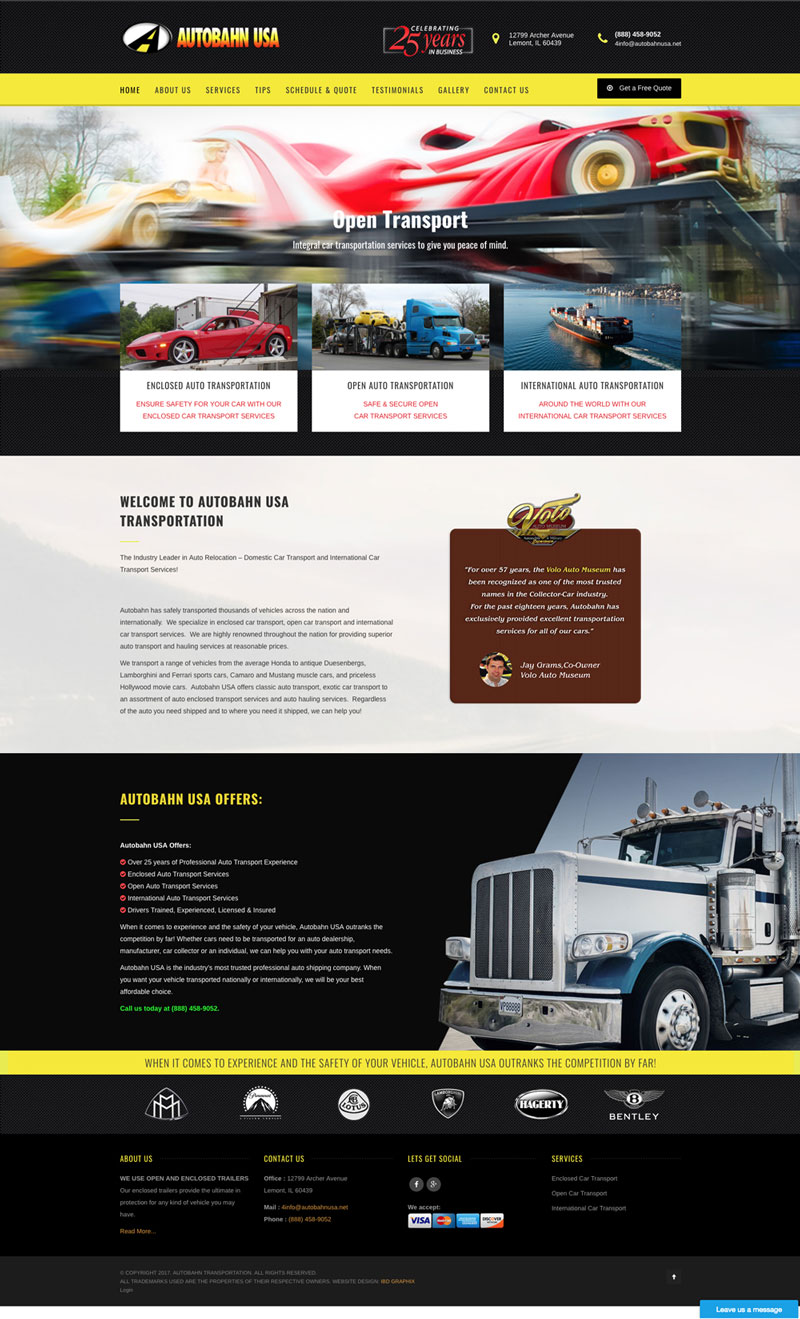**Detailed Descriptive Caption:**

The logo for Autobahn USA is prominently displayed, marking the company's 25th anniversary. Adjacent to the logo, a yellow bar contains text that is too small to decipher. Below, an image depicts a car on a trailer, labeled "Open Transport." Three additional images illustrate different vehicle shipping methods: one shows a car being loaded into a shipping container, another depicts a car being secured onto a big rig truck, and the third implies cars being transferred via boat.

Beneath these images, bold text reads, "Welcome to Autobahn USA Transportation," followed by an indistinguishable smaller text. There is a dark red-brownish box containing a probable thank-you message or a quote from the company's director, alongside a small image of a man in a suit with too-small-to-read accompanying text. 

Further down, another section features a big rig truck image on a black background with some gray text that remains unreadable. A subsequent yellow bar with legible text declares, "When it comes to experience and the safety of your vehicle, Autobahn USA outranks the competition by far."